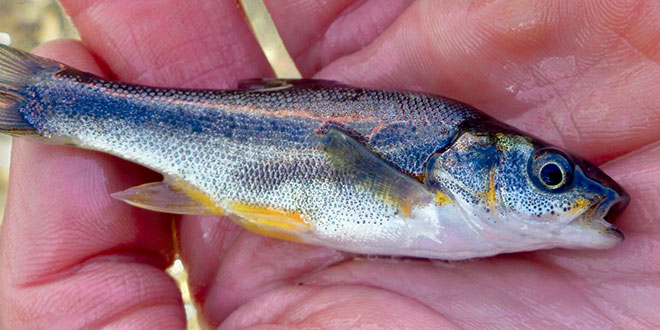The photograph showcases a close-up of a small fish held in the wet hand of a person, likely a Caucasian male. The fish, appearing freshly caught with glossy, wet scales, rests with its head to the right and tail to the left. Its body displays a striking combination of colors: a silvery-white belly, a speckled blue back, and yellowish fins and mouth. One open eye stares directly at the camera. Captured in natural sunlight, the detailed image allows us to observe the glistening scales and subtle hues of the fish, as well as parts of the person's thumb, index finger, and middle finger cradling it.